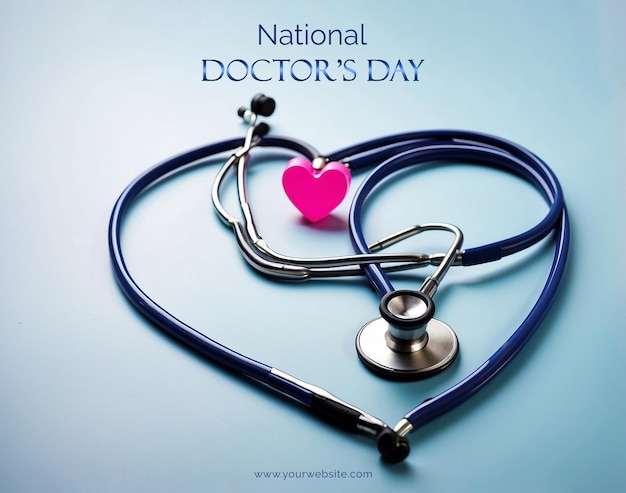The image is a detailed, digitally crafted graphic designed to celebrate National Doctors Day. Set against a blue-gray, aquamarine-colored background, the focal point is a silver and blue stethoscope artfully arranged into the shape of a heart. Positioned in the center of this heart shape is a pink, 3D Valentine's-style heart, adding a touch of warmth and symbolizing care and compassion. At the top of the image, in bold blue letters, is the text "National Doctors Day," acknowledging the occasion. At the very bottom, in small blue lowercase lettering, is the website address "www.yourwebsite.com," indicating that the image could be used for marketing or online purposes, possibly as a template for a medical website. The design is clean and simple, emphasizing the theme of appreciation for medical professionals.